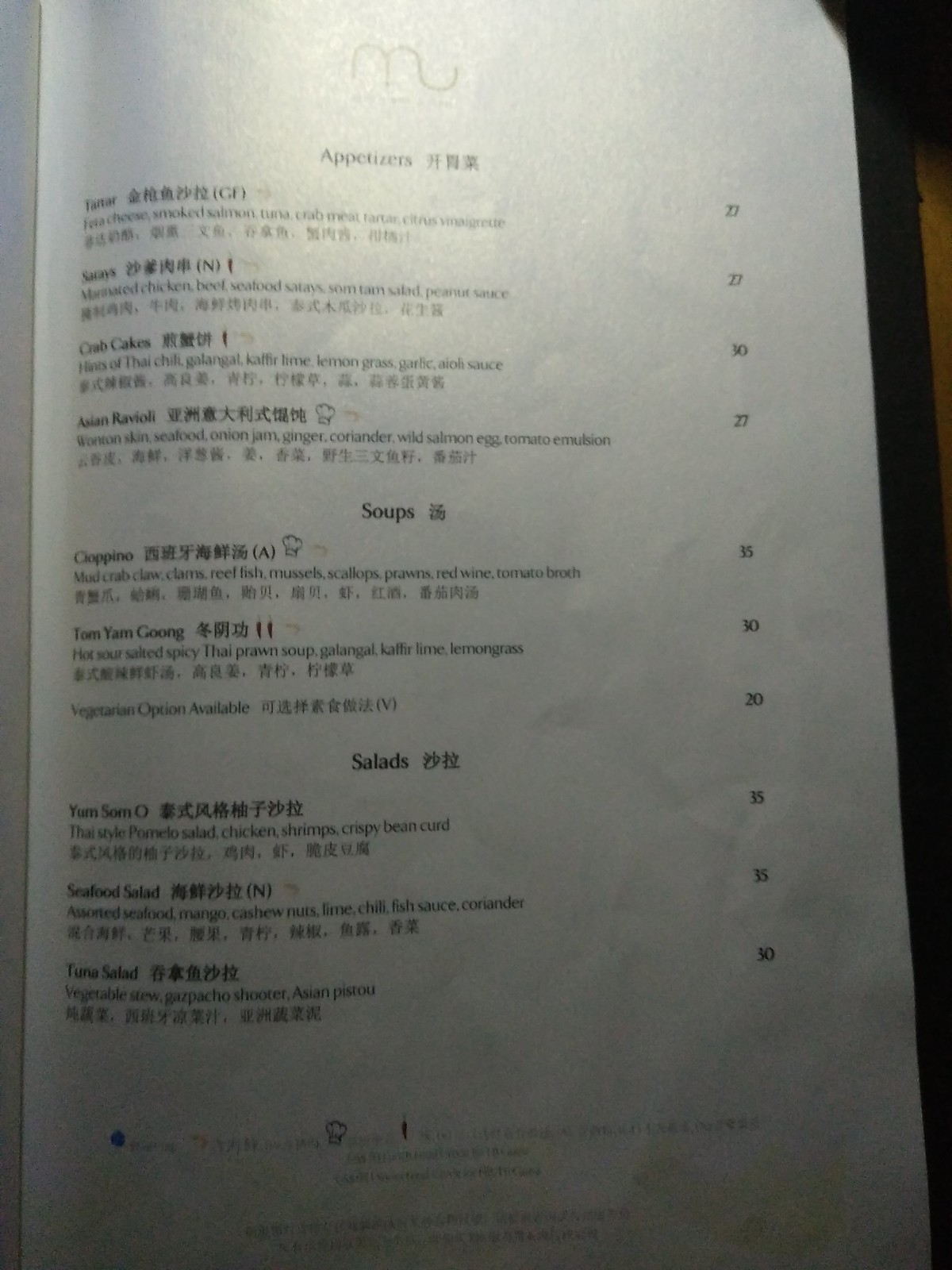The photo depicts a page from a restaurant menu, laying flat on a light wooden table. The menu has a thick, faux-leather cover that gives it a book-like appearance. The pages inside are white with plain black print, featuring a bilingual format in English and what seems to be Japanese characters.

The menu begins with a section labeled "Appetizers," offering options like crab cakes and Asian ravioli. Each dish description is followed by its price on the right. Next is the "Soups" section, where Tom Yum soup is notably listed. Following that, the "Salads" section features options such as seafood salad and tuna salad.

At the bottom of the page, though the text is not entirely legible, it seems to include the restaurant's name, phone number, website, address, and possibly some business registration or identification numbers.